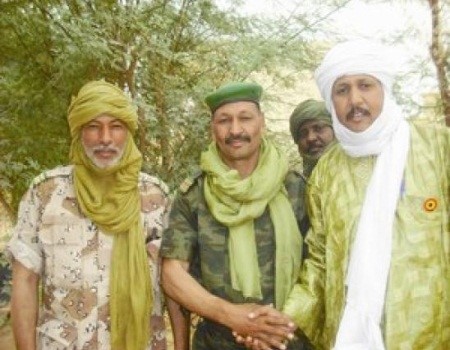In an outdoor setting, four Indian men stand in front of a backdrop of abundant green trees, capturing the essence of nature. The leftmost man is adorned in a beige short-sleeve shirt with a brown pattern, complemented by a mustard green Indian hat and a long scarf. Next to him stands another man wearing a dark green hat with a lime-colored folded scarf, clad in a short-sleeved, camouflage soldier uniform. The third man, slightly obscured and positioned behind the first two, showcases only his face, sporting a green Indian hat. The tallest man on the right wears a white Indian hat and a matching long white scarf, donning a lime green long-sleeve outfit with small orange and yellow accents. This group, amidst the towering trees and hints of a whitish sky, is central to the photograph, highlighting their traditional attire and unified presence in nature.